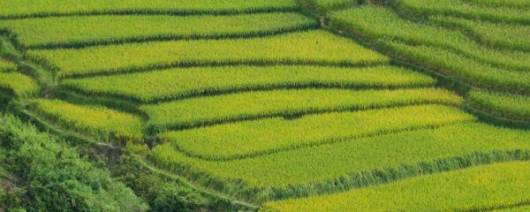This is a wide-angle, photorealistic image, slightly blurry or stylized, of extensive agricultural fields arranged in a horizontally aligned, tiered formation. The image, taken from a height, displays predominantly light green, rectangular fields that could be rice or a similar crop, bordered by darker green bands of vegetation. The scene extends horizontally from the bottom right, sloping up towards the top left, while the top right corner features fields with a more bowed, terraced structure sloping from the left to the right. On the left side of the image, a hill covered with rougher, wild shrubbery contrasts with the neatly manicured fields, indicating a transition from cultivated land to natural landscape. Similarly, to the right of the image, terraced steps of agricultural land ascend, maintaining the continuity of monoculture. The fields appear to be segmented by green hedges, adding to the pattern of the landscape. The overall appearance suggests an agricultural terrain with no visible machinery or people, captured in poor quality with slight focus issues.